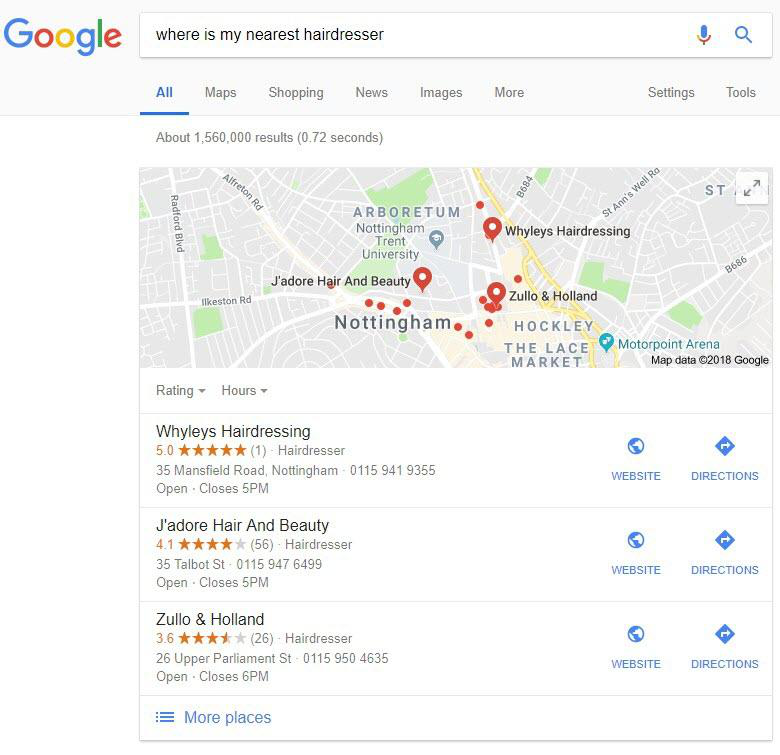This image is a screenshot of a Google search results page. The background is predominantly light, typical of Google's interface. In the upper left-hand corner, the Google logo is displayed, showcasing the familiar blue, red, yellow, and green color scheme of the letters. 

Below the logo is the search box stretching across the width of the image. The search term entered is "Where is my nearest hairdresser?" To the right of the search box, both the microphone icon and the magnifying glass search icon are visible.

Directly beneath the search box are several tabs that allow the user to filter search results, including "All," "Maps," "Shopping," "News," and "Images." The "All" tab is currently selected. Below these tabs, the search results indicate approximately 1,560,000 results found in 0.72 seconds.

The top search result displays a map of the local area, with red pins marking the locations of nearby hair salons. Below the map are corresponding listings that provide detailed information about each salon, including the name, rating, address, contact information, business hours, and links to the salon's website and directions.